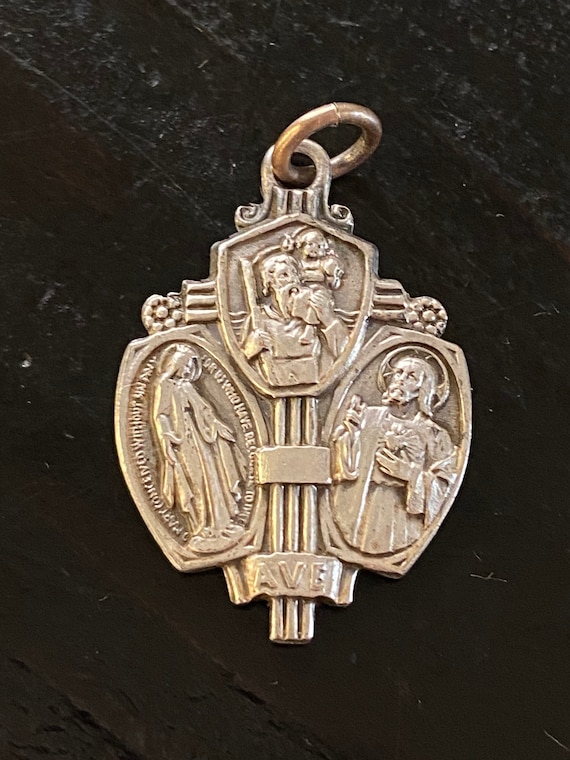This close-up photograph showcases an antique religious pendant, centered against a black marble-like background, characterized by its hints of grayish whitish veins. The pendant, appearing to be made of pewter with its dull silver hue, is small and structured in the style of a cross. At the top, a brass loop indicates its function as a component of a necklace. The pendant is divided into three distinct sections, each engraved with the image of a religious figure, likely depicting the Virgin Mary, Jesus, and God. The Virgin Mary is looking down and to her left, Jesus looks up and to his left, and God also looks up and to the left. Below these engravings, the letters "A-V-E" are inscribed, further emphasizing its religious significance.